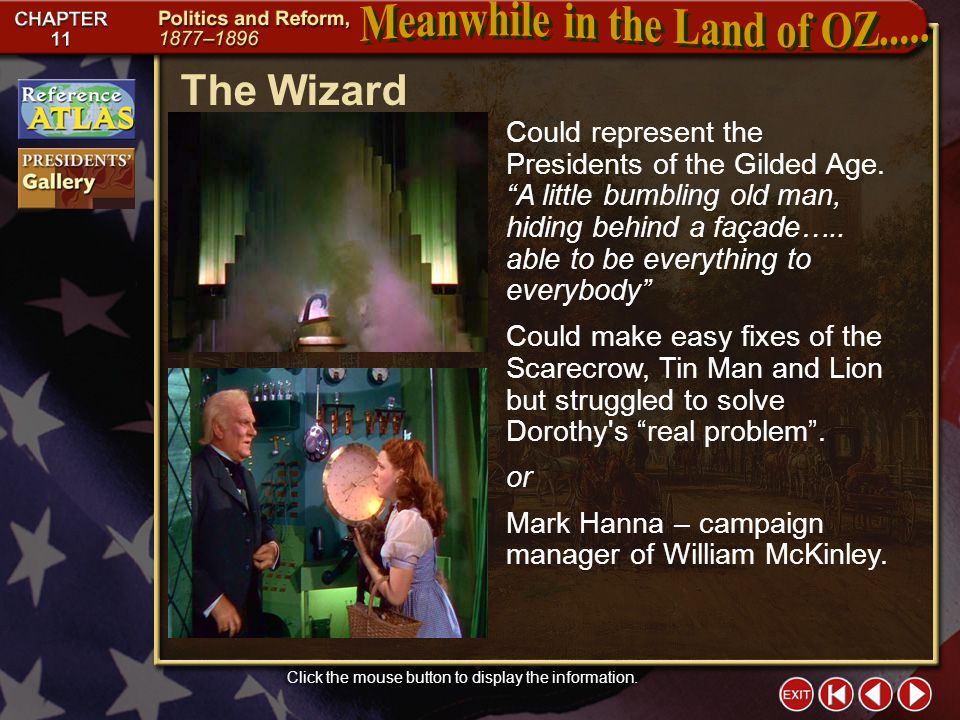The image is a slide from a PowerPoint presentation focused on the political landscape and reforms between 1877 and 1896, designated as Chapter 11. The background prominently features an American flag, symbolizing the nation's context during the Gilded Age. In the upper left corner, "Chapter 11" in bold red stands out, while the upper right corner displays the phrase "Meanwhile, in the land of Oz" in gold letters, linking the historical analysis to the iconic film.

The main content of the slide is framed within a brown square, over which various texts in different fonts are layered. At the top of this square, the title "The Wizard" appears in pale yellow font, directly tying the content to a character from "The Wizard of Oz." Below, in white text, it suggests that "the wizard could represent the presidents of the Gilded Age, a little bumbling old man hiding behind a facade, able to be everything to everybody," drawing a metaphor between the presidents of that era and the deceptive wizard character.

A new paragraph continues the analogy, stating that the wizard "could make easy fixes for the Scarecrow, Tin Man, and Lion but struggle to solve Dorothy's real problem," paralleling the superficial solutions offered by Gilded Age presidents. It also posits an alternative comparison of the wizard with Mark Hanna, the campaign manager of President William McKinley.

An inserted image further enhances this analogy, depicting an older white man conversing with Dorothy, evoking the dynamic between the wizard and other characters in the movie and illustrating the educational yet critical narrative presented in the slide.